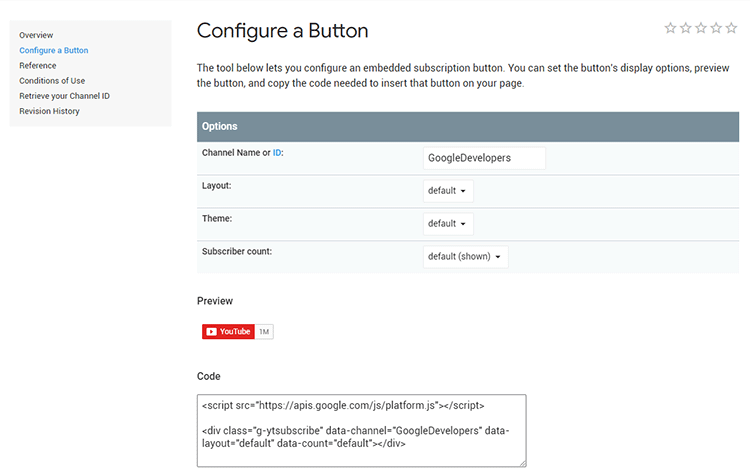This image is a screenshot of a web page taken from a desktop computer, specifically showcasing the "Configure a Button" page. The page features a small vertical scrollbar on the left-hand side with a menu listing options such as Overview, Configure a Button, Reference, Conditions of Use, Retrieve Your Channel ID, and Revision History.

In the main section of the page, the title "Configure a Button" is prominently displayed at the top left. To the top right corner, five empty star icons are visible. Below the title, the page explains, "The tool below lets you configure an embedded subscription button. You can set the button's display options, preview the button, and copy the code needed to insert that button on your page."

A gray banner labeled "Options" runs across the left-hand column, under which four configurative sections are outlined:

1. "Channel Name or ID" with "Google Developers" selected.
2. "Layout," which features a default scroll option.
3. "Theme," also featuring a default scroll option.
4. "Subscriber Count," similarly with a default shown scroll option.

Below these sections, the page offers a "Preview" of what the button will look like, including a YouTube logo. At the very bottom is a "Code" section that displays the necessary script code in small black text, ready to be copied for embedding the button.

The overall design features ample white space, especially noticeable at the bottom-left side and the right bottom corner of the page, giving it a clean and uncluttered look.